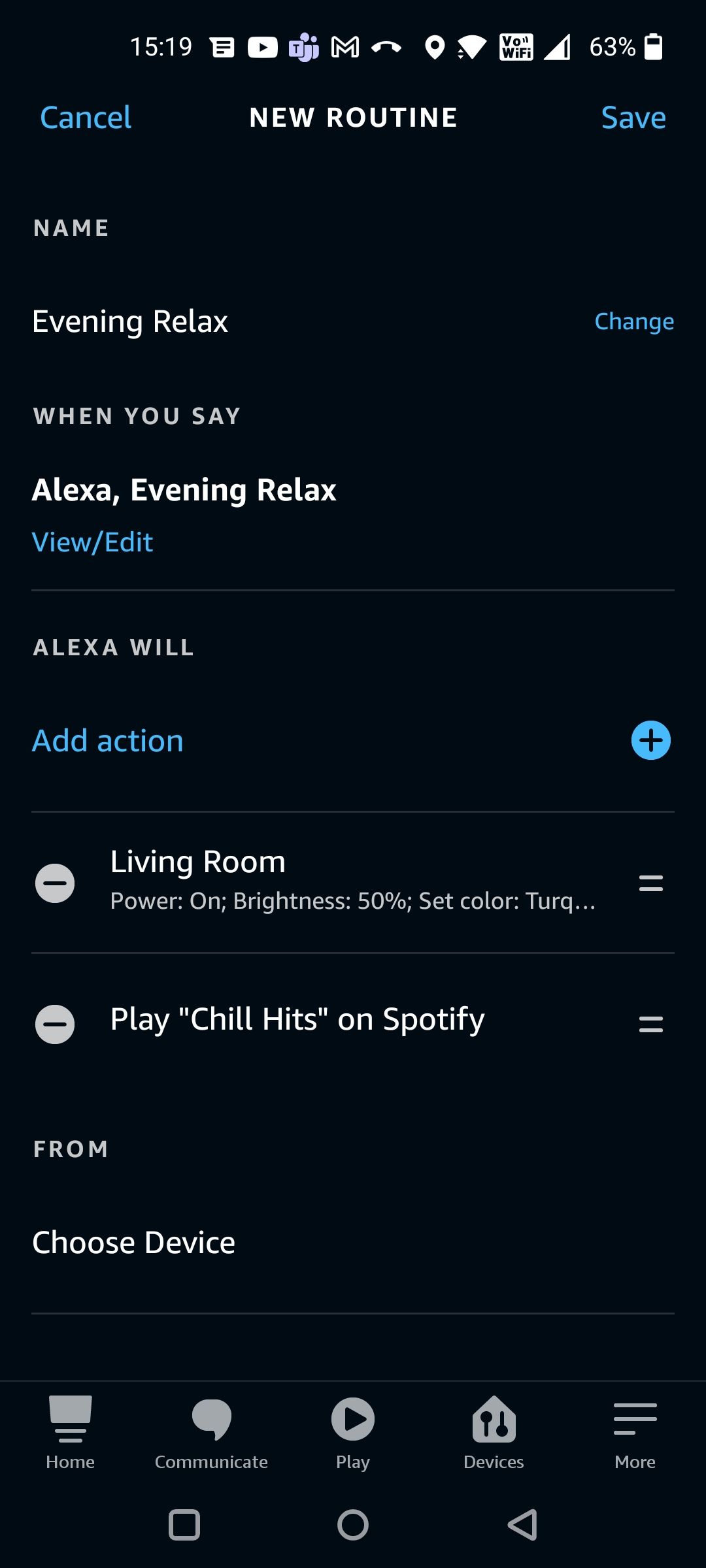The color photograph captures a vertical screenshot of a smartphone display. At the top of the screen, standard icons display various statuses: the time reads 15:19, the battery level is at 63%, and the signal strength and network indicators are clearly visible along with the Wi-Fi status.

Just below, the screen displays bold, uppercase text in white reading "NEW ROUTINE," flanked by options in light blue text on either side: "Cancel" on the left and "Save" on the right. Further down, the label "NAME" is prominently shown in capitalized white text, followed by the editable field “Evening Relax, Change.”

The next section, "When you say," precedes the phrase "Alexa, Evening Relax," underlined by an option in blue text reading "View/Edit." A thin horizontal line separates these sections from the following part, where gray text declares "ALEXA WILL." In light blue text, with an accompanying black plus sign within a bubble, is the prompt "Add Action."

Below this, the specified action reads “Living room,” followed by the instruction “Play Chill Hits on Spotify from choose device,” indicating the desired music and device settings for the routine.